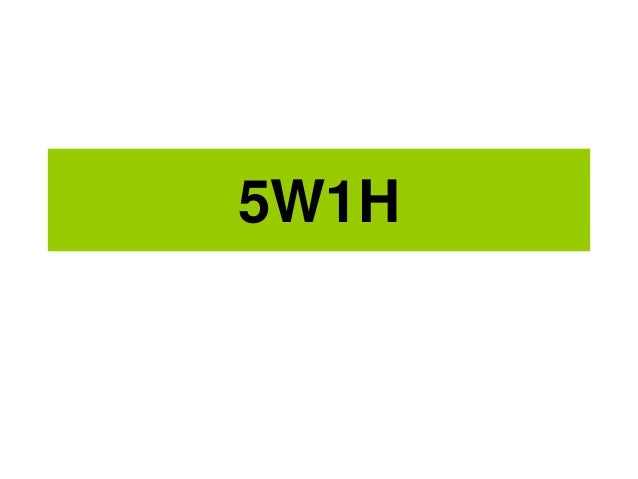The image features a light or lime green rectangular box with a solid background and no outline, resembling an avocado green shade. Centered both horizontally and vertically within this green rectangle is an alphanumeric sequence, "5W1H," rendered in a black, sans-serif font similar to Arial. The sequence consists of the number 5, an uppercase W, the number 1, and an uppercase H, collectively occupying the central space of the rectangle like a concise license plate.